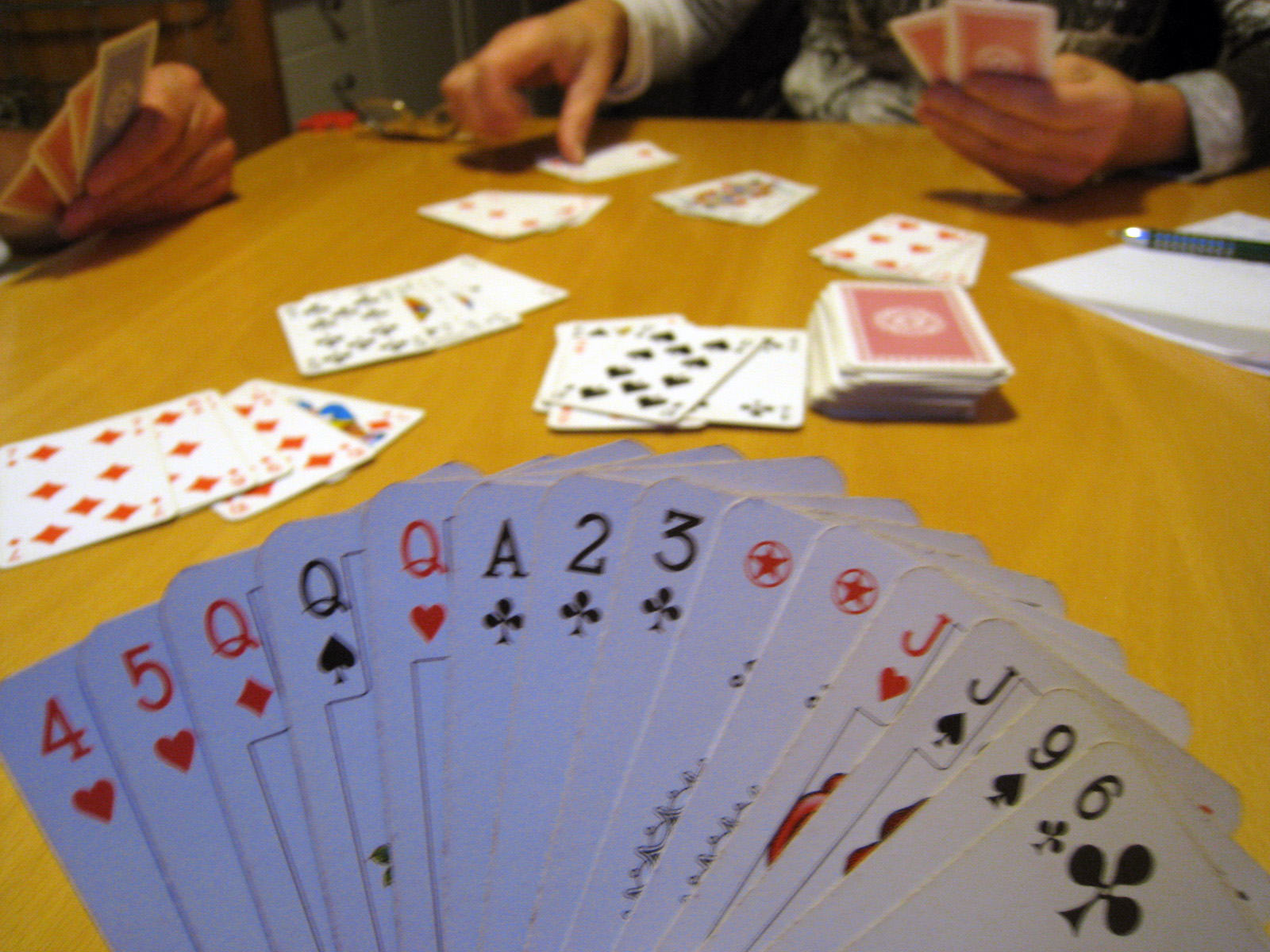In this indoor digital photograph of a poker game, various elements of the scene are captured in detail. 

In the upper left corner, a Caucasian hand is seen holding a fan of red and white playing cards. On the right side, a person is partially visible, dressed in a long white-sleeve shirt layered under a short-sleeve black shirt. This individual has one hand on the table, touching a white playing card, suggesting they might be the dealer. 

Beneath their hand, there is a folded white piece of paper with a black pen placed on it, its silver tip catching the light. The playing table itself is made of light tanned wood, adding warmth to the scene.

At the center-right of the table, a neatly stacked pile of cards is positioned alongside some flipped-over cards. The prominent card on top is the black eight of hearts. Other sprawled cards, slightly obscured, hint at a variety of diamond cards.

A main hand in the frame holds a large assortment of playing cards. Visible among them are the red four of hearts, the red five of hearts, the queen of diamonds, the queen of spades, the queen of hearts, and the ace of clubs. Also seen are the two and three of clubs, a card with two red stars and a red circle, the jack of hearts, the jack of spades, the black nine of spades, and the six of clubs.

The detailed array of cards, coupled with the individuals and the setting, vividly captures the intensity and focus of the poker game.